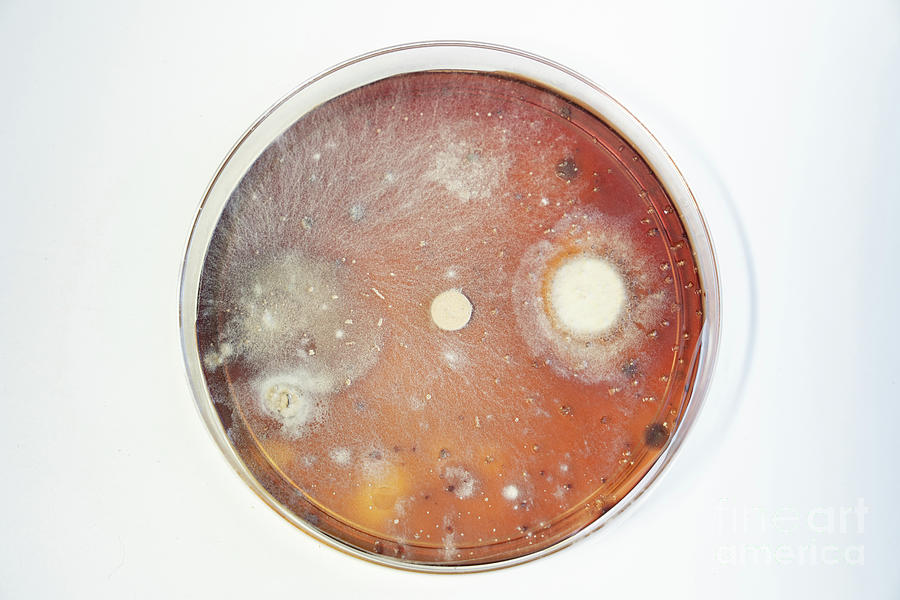This is a top-down photograph of a circular Petri dish placed on a white surface, likely taken in a light box. The dish is made of glass with a silver rim and contains a dark reddish-brown liquid. Within this liquid, there are various substances including gray and white particles distributed throughout. Specifically, on the right side, a prominent white circular colony can be seen, while on the left, gray spread-out particles are visible. Scattered bubbles are present along with a different range of fuzzy, stringy fungal growths and multiple whitish bacterial colonies. There is a faint watermark in white at the lower right corner of the image, which appears to say "art america," though it's barely legible against the white background.